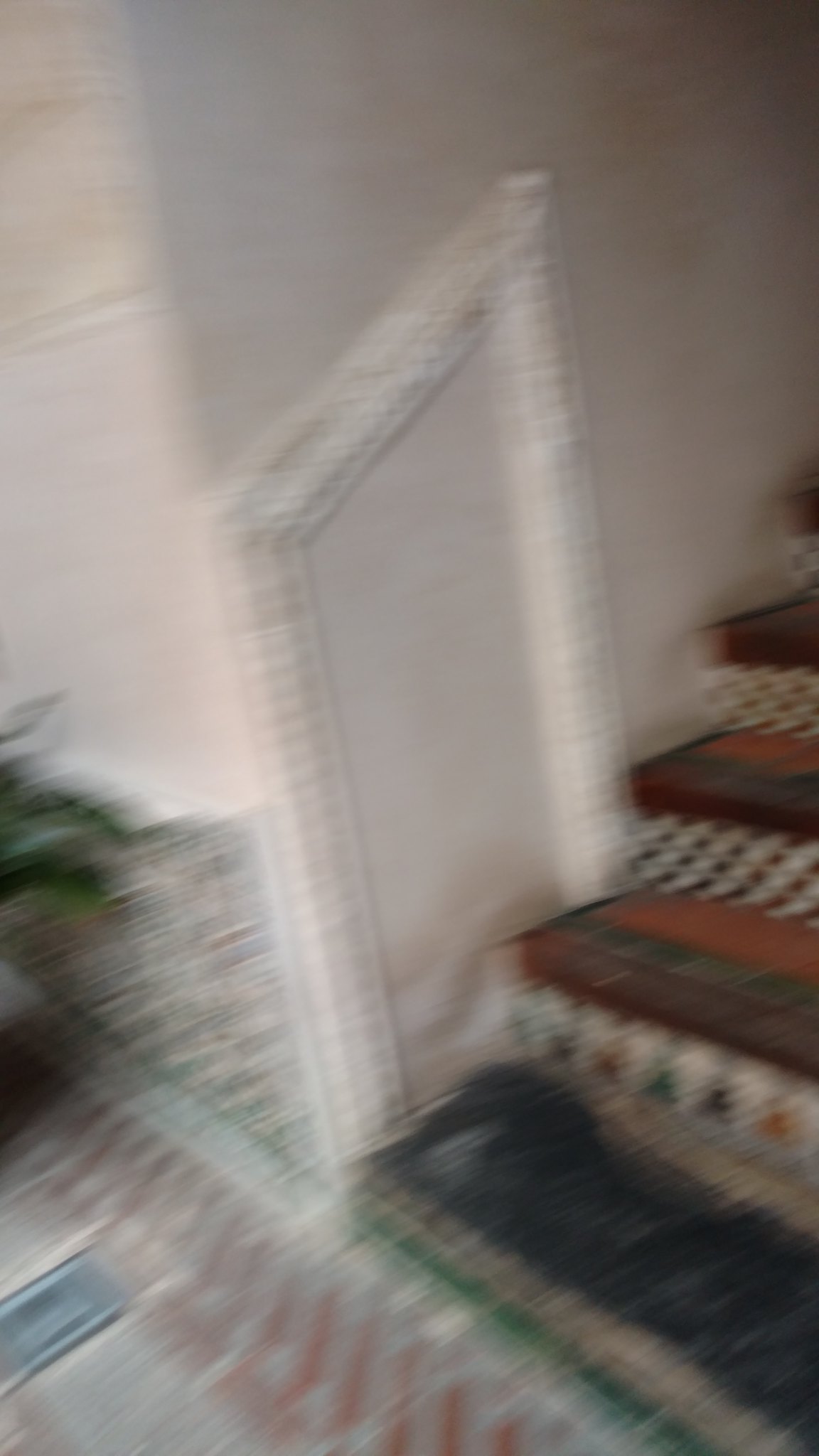This is an out-of-focus photograph, likely taken inside someone's home in motion. At the bottom left, there is a striped carpet with red, green, possibly blue, and white patterns. The background wall is pink with white trim at the base, and each step of the stairway features a black and red coloration with various painted patterns such as checkers, triangles, and images in different colors like yellow and green. To the right of the image, the stairway ascends with each step adorned in colorful carpets featuring varied designs and hues. The left center of the image reveals a green leafy plant, while a light gray wall with a white picture frame (empty) is also visible. Additionally, a floor vent can be seen near the plant before the stairs begin. Despite the blurriness, the vibrant, eclectic decor and intricate stair patterns are notable.